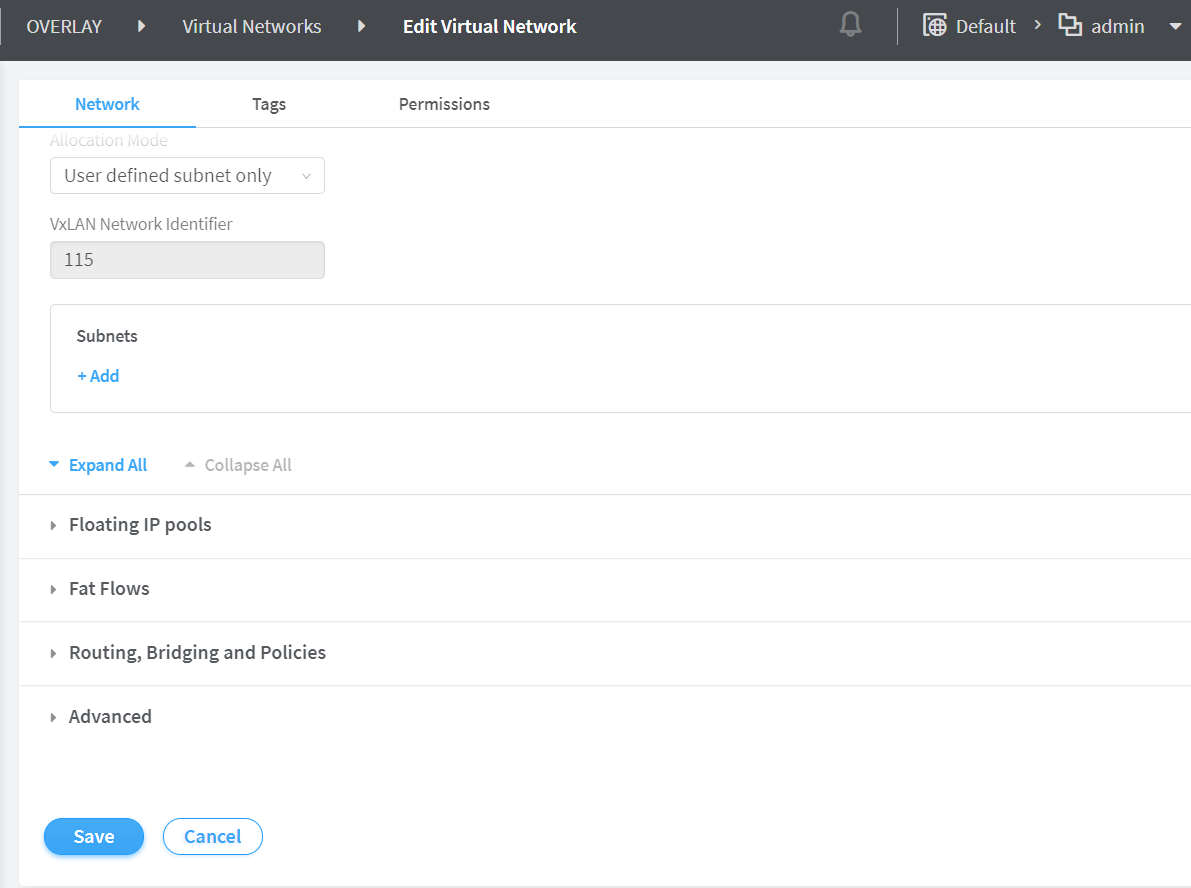The image displays a digital interface, potentially an application, program, or website, characterized by its detailed navigational and functional layout. The aspect ratio of the image is approximately 20% wider than it is tall. 

At the very top of the interface, there is a black header bar with white text, detailing three navigational areas: "Overlay," "Virtual Networks," and "Edit Virtual Network," each separated by a right-pointing arrow. The last navigational area, "Edit Virtual Network," is bolded, indicating it is the active selection. Adjacent to this is a grayed-out alert icon and two drop-down menu options labeled "Default" and "Admin."

The main area of the interface features a white background and is divided into three horizontal tabs: "Network," "Tags," and "Permissions." The "Network" tab is currently active, marked by bold text with a blue underline. Below these tabs, the interface offers different options, starting with a drop-down menu labeled "User Defined Subnet Only."

Further down, there is a section titled "VXLAN Network Identifier" containing a gray box with the number "115" displayed inside it. Continuing downward, the section titled "Subnets" is bolded, followed by light blue text that reads "+ Add," suggesting the option to add new subnets.

Overall, the interface is structured with clear sections and options, allowing for detailed network configuration and management.